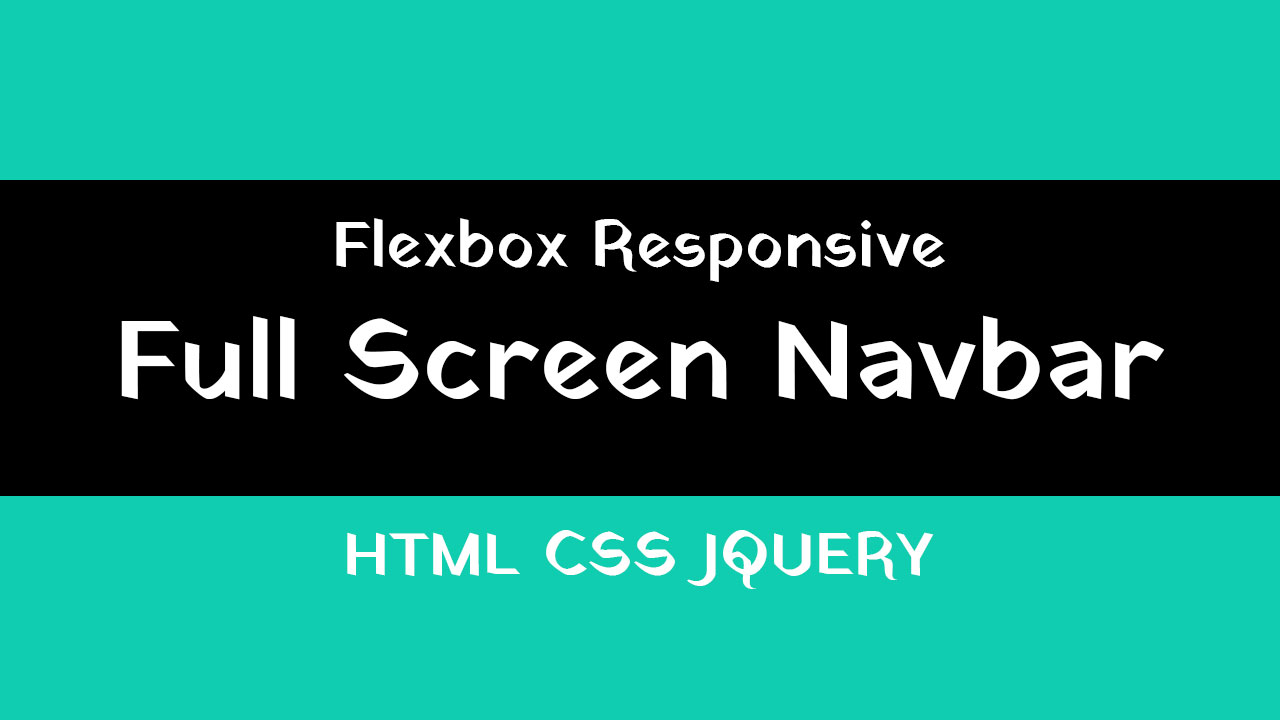This image features a turquoise background with a central black bar containing white text. The text on the black bar reads, "Flex Box Responsive Full Screen Nav Bar" in a clear, sans-serif font. Below the black bar, within the turquoise area, the terms "HTML," "CSS," and "jQuery" are prominently displayed in uppercase letters. Additionally, there is a calligraphy-style script that reads "http://www.kenhub.com," providing a refined contrast to the otherwise modern, straightforward typography. The overall design appears to be a sophisticated advertisement or promotional content for web development solutions.